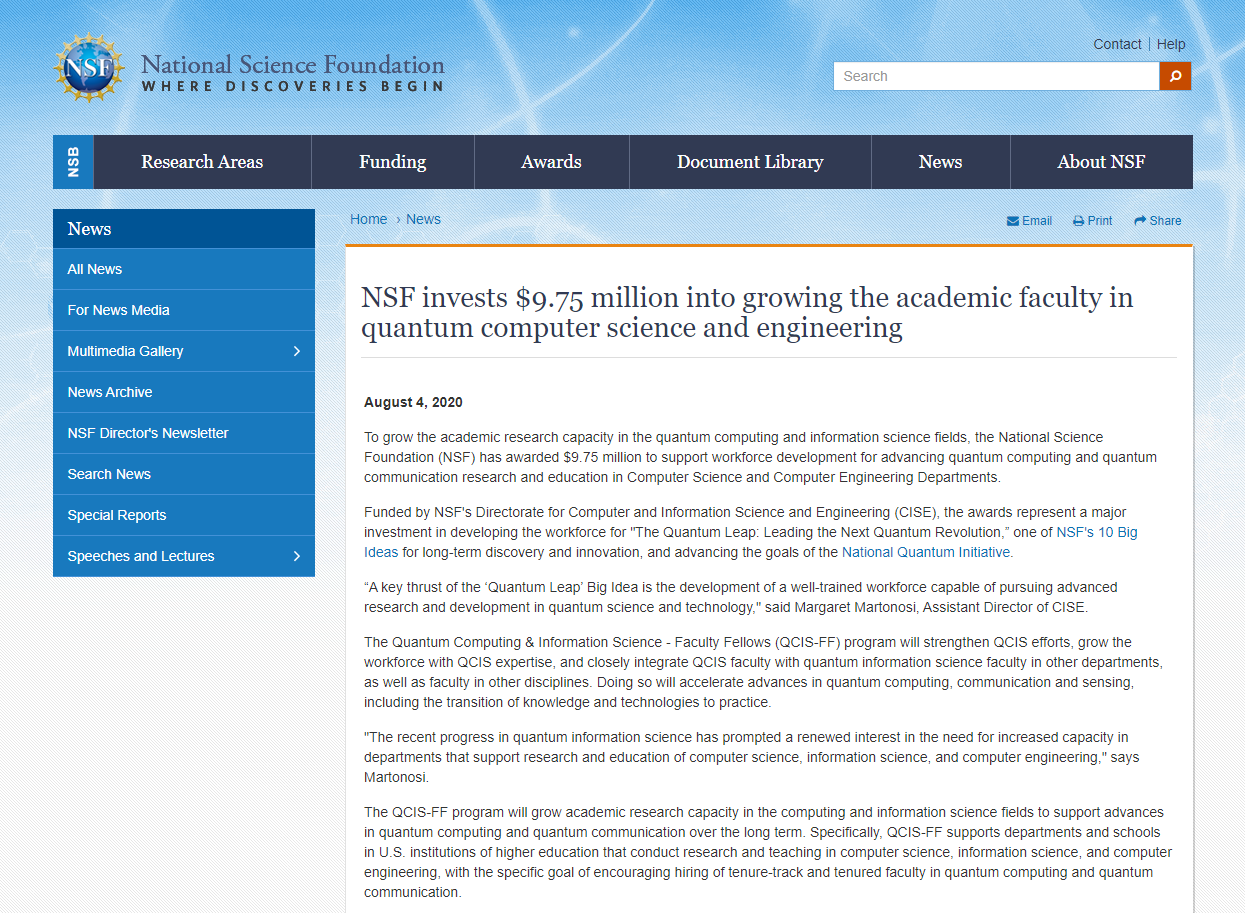**Detailed Caption:**

The screenshot captures a webpage from the National Science Foundation (NSF), prominently featuring their tagline "Where Discoveries Begin." The page header includes a search bar on the top-right corner, with navigational links for "Contact" and "Help" above it. A horizontal black menu bar beneath the header lists various areas of the site, including NSB, Research Areas, Funding, Awards, Document Library, News about NSF, Email, Print, Share, Home, and News.

To the left, a vertical menu offers specific navigation options such as News, All News, Fox News Media, Multimedia Gallery, News Archive, NSF Director's Newsletter, Search News, Special Reports, Speeches, and Lectures.

The main body of the image contains an announcement dated August 4th, 2020, detailing NSF's $9.75 million investment aimed at expanding the academic faculty in quantum computer science and engineering. The objective is to enhance research capacities in quantum computing and information science through workforce development, supporting the advancement of these fields in computer science and computer engineering departments. This funding is provided by NSF's Directorate for Computer and Information Science and Engineering (CISE).

The announcement highlights the award's aim to further the NSF's "Quantum Leap" initiative—part of its 10 big ideas for long-term discovery and innovation—and to advance the National Quantum Initiative's goals. The initiative is focused on cultivating a highly trained workforce to drive forward quantum science and technology.

Margaret Martonosi, NSF's CISE Assistant Director, is mentioned as the presenter of the award. The Quantum Computing and Information Science Faculty Fellows (QCIS-FF) program is specifically designed to enhance QCIS endeavors, grow expertise in the field, and foster integration among quantum information science faculties within their respective departments and other disciplines. This integration aims to expedite advancements in quantum computing, communication, and sensing technologies.

Martonosi underscores the increasing need for departmental capacity to support quantum information science research and education, driven by recent scientific progress. The QCIS-FF program targets U.S. higher education institutions, providing them with support to hire tenure-track and tenured faculty specializing in quantum computing and quantum communication, ensuring sustained advancement in these cutting-edge fields.